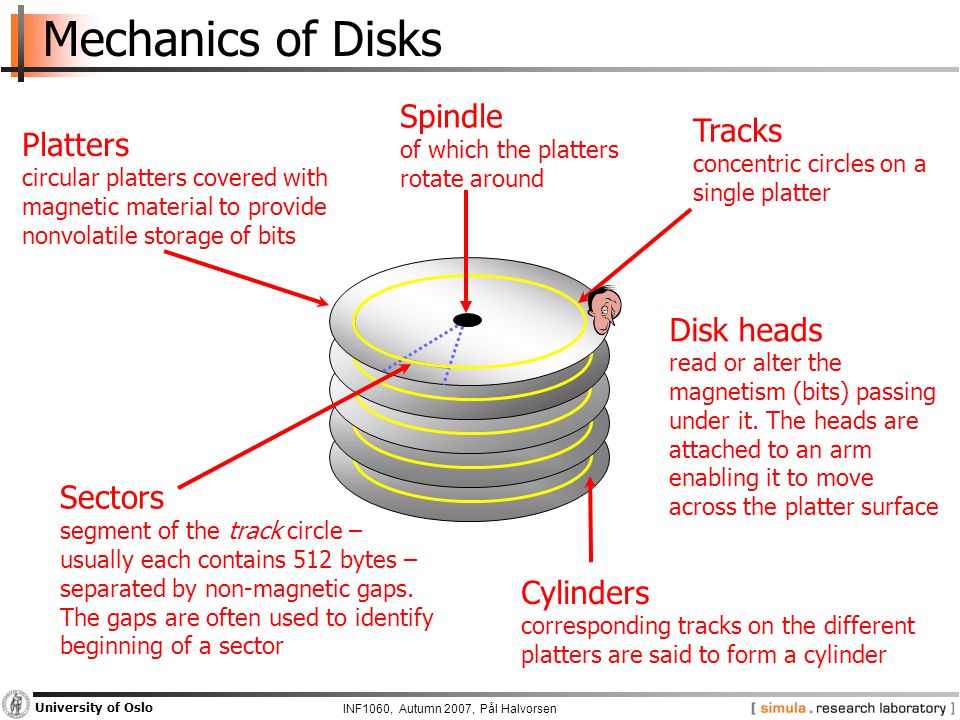The PowerPoint slide features a detailed educational diagram titled "Mechanics of Discs" on a solid white background with a black headline and an orange shaded square next to the 'M.' At its center, a stack of five silver disks is illustrated, encircled by red text and arrows pointing to various parts of the disks. These parts include platters, spindles, tracks, disc heads, cylinders, and sectors. The disks have yellow circles, with a blue perforated line marking a sector, accompanied by a red arrow and descriptive text explaining that a sector is a segment of the track circle containing 512 bytes. The platters are circular and covered with magnetic material for non-volatile storage, while the spindle refers to the axis around which the platters rotate. Tracks are described as concentric circles on a single platter. The cylinders represent corresponding tracks across multiple platters. At the bottom of the slide, a black line contains text designating the University of Oslo, INF 1060, Autumn 2007, and the researcher P. Pal Haverson from Simula Research Laboratory. The overall style of the slide is illustrative and educational, intended for academic use.